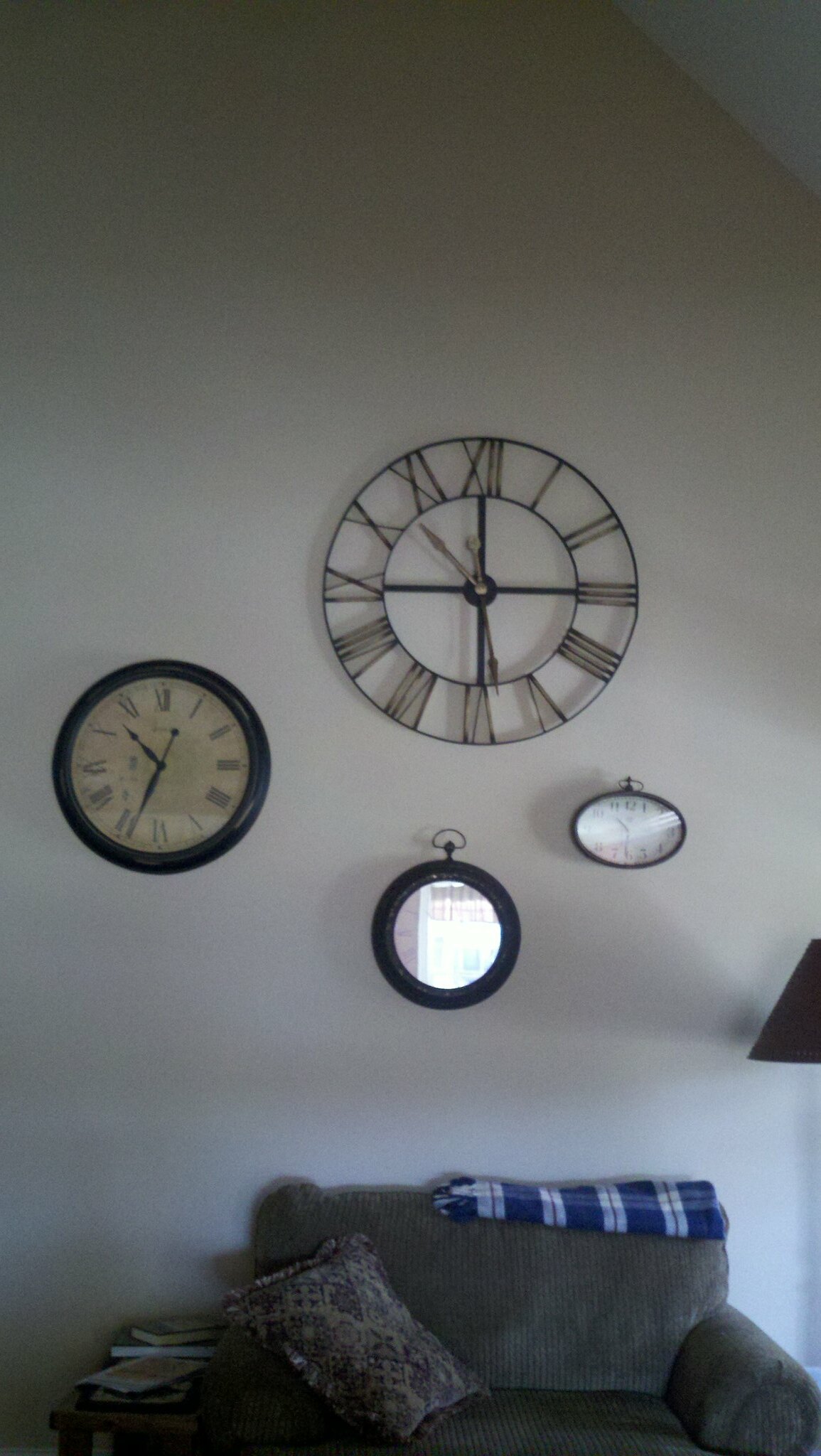The image depicts a section of a predominantly white wall in a house adorned with four distinct wall hangings. Three of these hangings are clearly clocks, and the fourth, obscured by a strong reflection likely caused by a nearby window, may also be a clock. 

On the left side of the wall is a vintage clock characterized by a solid black outline. This old-fashioned timepiece features Roman numerals and has a black and white design with a tan clock face, all encased under a glass cover.

Centrally positioned at the top is a unique wireframe clock. This clock showcases an intricate open design with a black wire structure and gold hands that attach at a T-shaped cross pattern in the center. The clock also displays Roman numerals along its circumference.

On the bottom right, there is a small, sideways oval-shaped clock. Unlike the previous two, this clock uses standard numerical digits instead of Roman numerals.

Below these clocks is a comfortable, oversized gray chair with a blanket draped over its back. Adjacent to the chair is a stack of books resting on a side table, completing the cozy setting.

The overall ambiance suggests a blend of vintage charm and modern simplicity, highlighted by the interplay of natural light and reflective surfaces.